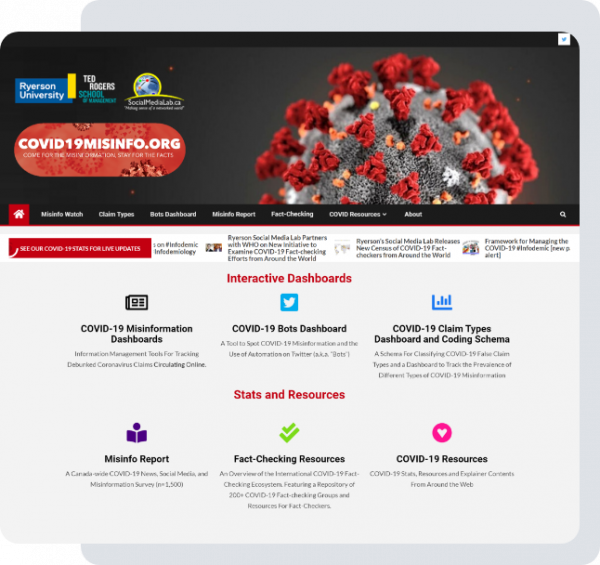In this screenshot, we observe a user interface set against a black background. Dominating the right side of the image is a detailed, scientific illustration resembling a magnified spore or germ. This circular, gray entity has a spongy texture, adorned with small red tree-like structures and orange dots scattered across its surface.

In the upper right corner, the Twitter bird logo is prominently displayed within a white box. Directly to its left, an orange button labeled "COVID-19missinfo.org" draws attention. Positioned in the upper left corner, there's a blue box containing the text "Ryerson University," adjacent to a black box that reads "Ted Rogers School."

Below these elements, on the left side of the image, a red button with white text invites users to "See our COVID-19 stats from live updates." In the center, bold, red text highlights "Interactive Dashboards." Further down on the left, the text "COVID-19 Misinformation Dashboards" is visible. 

To the right of these descriptions, several dashboard options are listed. They include the "Twitter Bird COVID-19 Bots Dashboard," which is described as a tool to identify COVID-19 misinformation and automated Twitter activity. Adjacent to this is the "COVID-19 Claim Types Dashboard and Coding Schema."